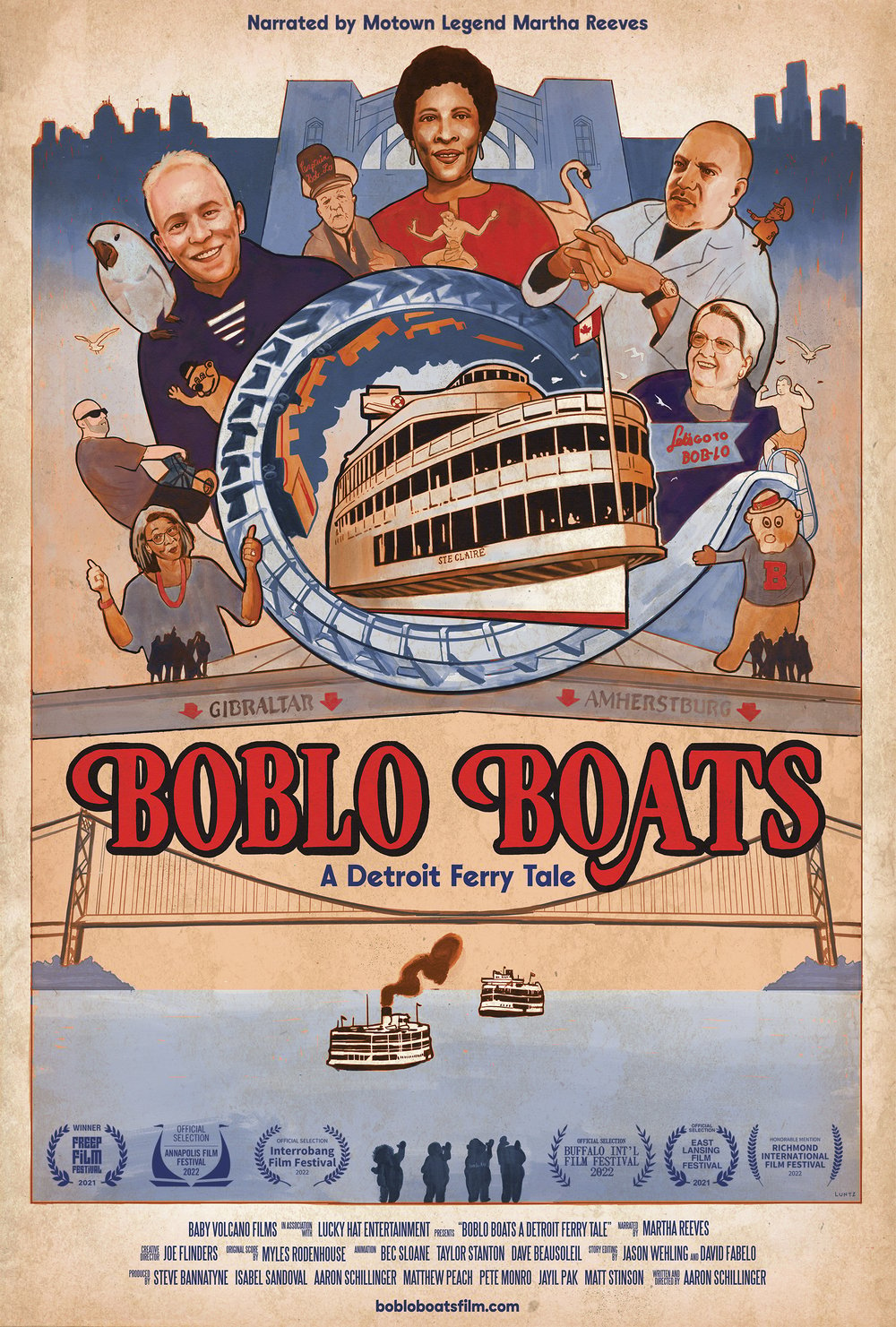This image is a detailed, vintage-style promotional poster for the movie "Boblo Boats: A Detroit Fairy Tale," narrated by Motown legend Martha Reeves. At the top of the poster, the title is prominently displayed. Above the title, there is an image of a fairy adorned with a Canadian flag, surrounded in a circle-based pattern by various characters from the movie, including a man with a cockatoo or a parrot on his shoulder and a mascot pointing at the fairy with his right hand, topped with a hat. The top section also features a large vintage steamship, indicative of the historical transportation theme. Below the title, the bottom part of the poster showcases a bridge spanning a bay, with two vintage steamships emitting steam as they navigate the waters. The poster also includes a promotional website, BobLoweBoatsFilm.com, offering additional details. This intricately designed poster beautifully captures the essence of the movie's historical and fantastical elements.